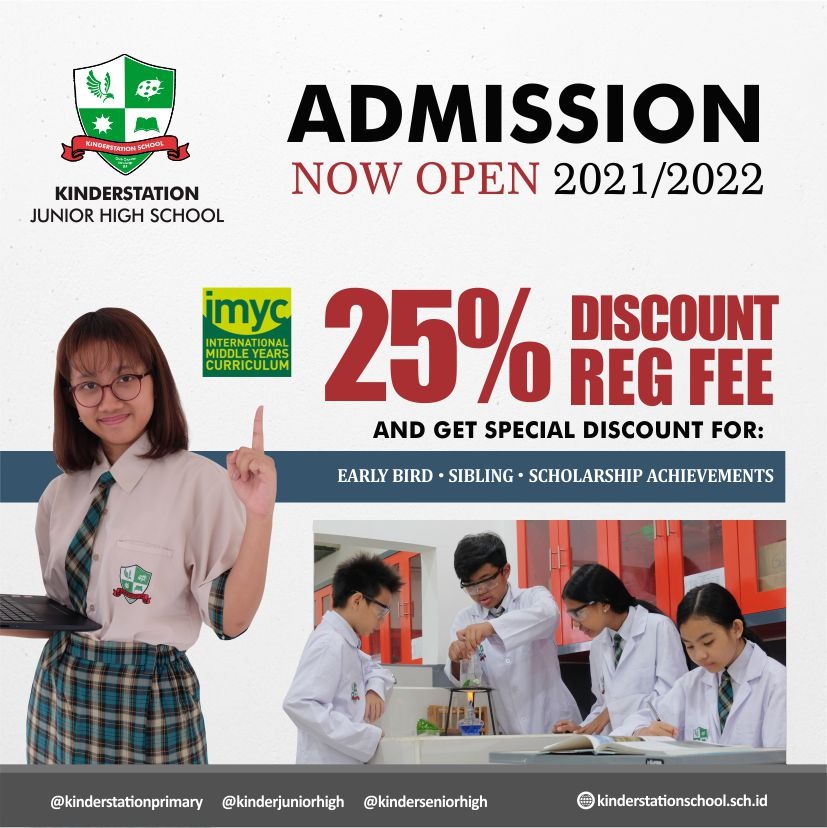This image is a detailed screenshot with a light gray, off-white background. Dominating the top left corner is a heraldic shield divided into four sections, each containing a distinct symbol: the upper left features a white background with a green eagle, the upper right showcases a green background with a white paint palette, the lower left displays a green background with a white sun, and the lower right has a white background with a green open book. Below the shield, a red ribbon runs horizontally, and beneath this ribbon, bold black text reads "Kinder Station," followed by "Junior High School," also in black and centered.

To the right of this shield, large, black, bold block letters spell out "ADMISSION." Directly underneath, in red, all caps, it states "NOW OPEN," and further down in black text, the years "2021/2022" are displayed.

On the left side of the image, there is a photograph of a young girl with shoulder-length dark hair and bangs. She wears dark glasses, a short-sleeve white button-down shirt, a green and yellow checkered tie, and a matching skirt. A dark gray rectangle spans behind her shoulders, and within this rectangle, white text reads "Early Bird Sibling Scholarship Achievements." 

Below this, another photograph depicts a group of children, all with dark hair. Some of them are wearing glasses, and they are all clad in white lab coats, seemingly engaged in a lab experiment.